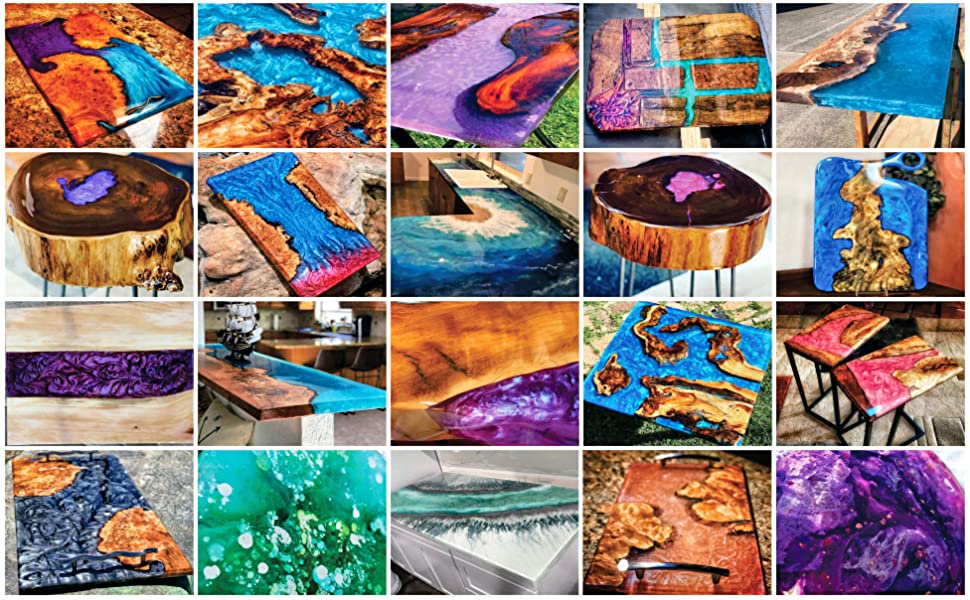The image features a grid of 20 color photographs depicting a variety of resin artworks, arranged with five photos in each row and four in each column. These artworks encompass both canvases and furniture, primarily coffee tables, employing a vibrant palette of purple, blue, light blue, pink, and deep aquamarine.

Prominently, there are several pieces resembling sections of tree trunks, one with a polished, glossy surface and a striking purple splotch in the center. Similarly, a table invoking the imagery of a shoreline shows a mix of wood and blue resin, mimicking coastal landscapes. Another piece displays a square wooden surface with intricate turquoise resin lines, reminiscent of river currents. Other notable images include a purple blob-like shape at the bottom right, and a piece on the top right that features brown tones with blue resin, invoking a naturally eroded look.

Overall, the array of photos seems to capture the surreal beauty of resin art, blending organic wood elements with vividly colored resins to create pieces that evoke natural scenery and abstract patterns.